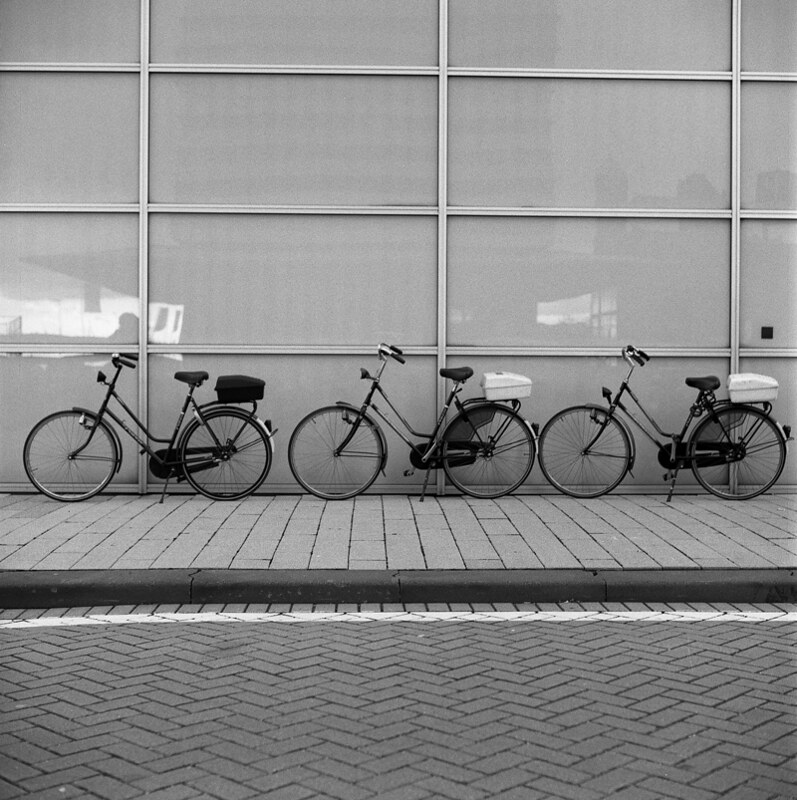The black-and-white photograph features three old-fashioned bicycles in a row on a stone sidewalk, adjacent to a brick roadway. The bicycles, which are nearly identical, feature high handlebars, large comfortable seats, and practical frames designed for easy city riding. Each bike has both front and rear lights, headlamps, chain guards, mudguards, and kickstands. Behind the seats, each bicycle is equipped with a carrier rack holding small storage containers; two bikes have white containers and one has a black container, resembling lunchboxes. They are positioned against a glass-walled building with rectangular criss-cross frames and windows covered by a white fabric, contributing to the overall gray tone of the scene.